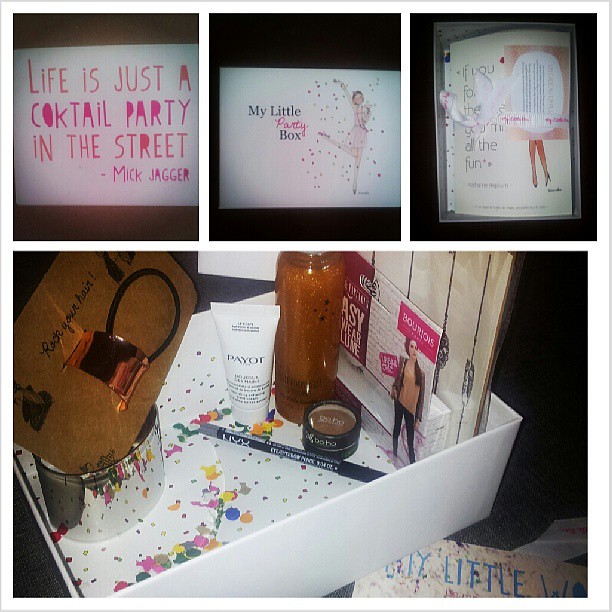This image features a vibrant and playful collage promoting a party-themed subscription box. The top row of the collage showcases three small images, each contributing to the party vibe. The left image displays a quote in pink text: "Life is just a cocktail party in the street," attributed to Mick Jagger. The center image highlights a jubilant woman in a pink dress with confetti all around her, captioned "My Little Party Box." The right image shows a card, possibly part of the box contents.

The larger image at the bottom of the collage reveals the subscription box itself, open to display various beauty products nestled among a festive confetti design. Items visible include a hair tie, hand jewelry, eyeshadow, lip liner, mascara, and skincare squeeze bottles, all arranged to emphasize the variety and delight of the box. The background is white, adding a clean and appealing contrast to the colorful contents. The overall aesthetic is fun, celebratory, and geared towards women looking to treat themselves.